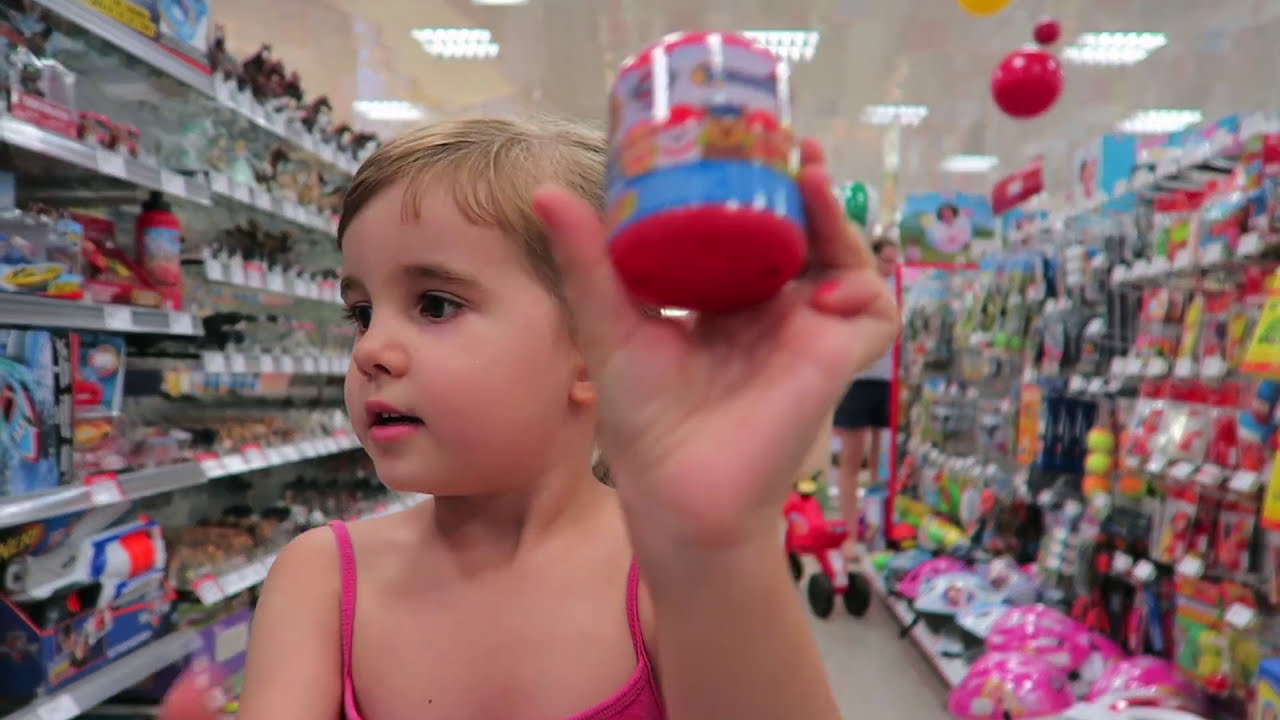The image captures a scene in the toy aisle of a large store, featuring a little girl with short blonde hair in the foreground. She is wearing a pink tank top with thin spaghetti straps and is standing with her body facing left while looking to her right. The girl's left hand, adorned with pinkish nail polish, is raised in front of her, holding a container that appears to have a pink base and blue details—possibly a tub of Play-Doh.

Surrounding her, the aisle is lined with a variety of toys and craft items. On her left, the shelves are densely packed with toys, including what looks like a toy Nerf gun and various art supplies such as paint and possibly nail polish. On her right, more items are displayed, though they are somewhat out of focus; the discernible items include tassels and small balls. The floor nearby holds a red ride-on toy with two wheels in the back.

In the background of the aisle, an adult dressed in a white shirt and dark shorts can be seen, adding a sense of scale and context to the environment, which has a white ceiling with many lights illuminating the space.